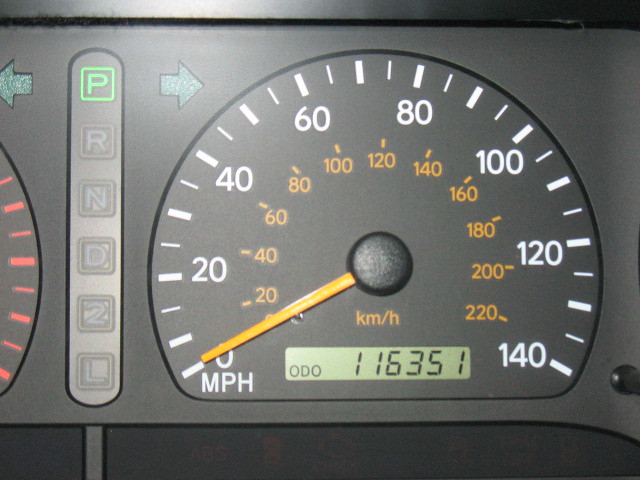This close-up photograph showcases the intricate details of a vehicle's instrument cluster. Dominating the frame is an analog speedometer with a bold red pointer. The dial displays speed in both miles per hour (mph) and kilometers per hour (km/h); the mph readings are marked in white against a black background, while the km/h are subtly indicated in orange. Illuminated for visibility in low light, the dial is complemented by a black center button.

Beneath the speedometer, a digital odometer (ODO) reads 11,635.1 miles, providing an exact mileage count. Adjacent to this digital readout, a transmission indicator bar is visible, backlit to show the current gear position—PRND2L, covering park, reverse, neutral, drive, second gear, and low gear options.

Additional elements in the image include the left and right turn signal indicators. To the left edge of the frame, another analog gauge is partially visible, hinting at either a fuel level, temperature gauge, or a more sophisticated tachometer for monitoring the engine's RPM, suggesting the vehicle's high-end features.